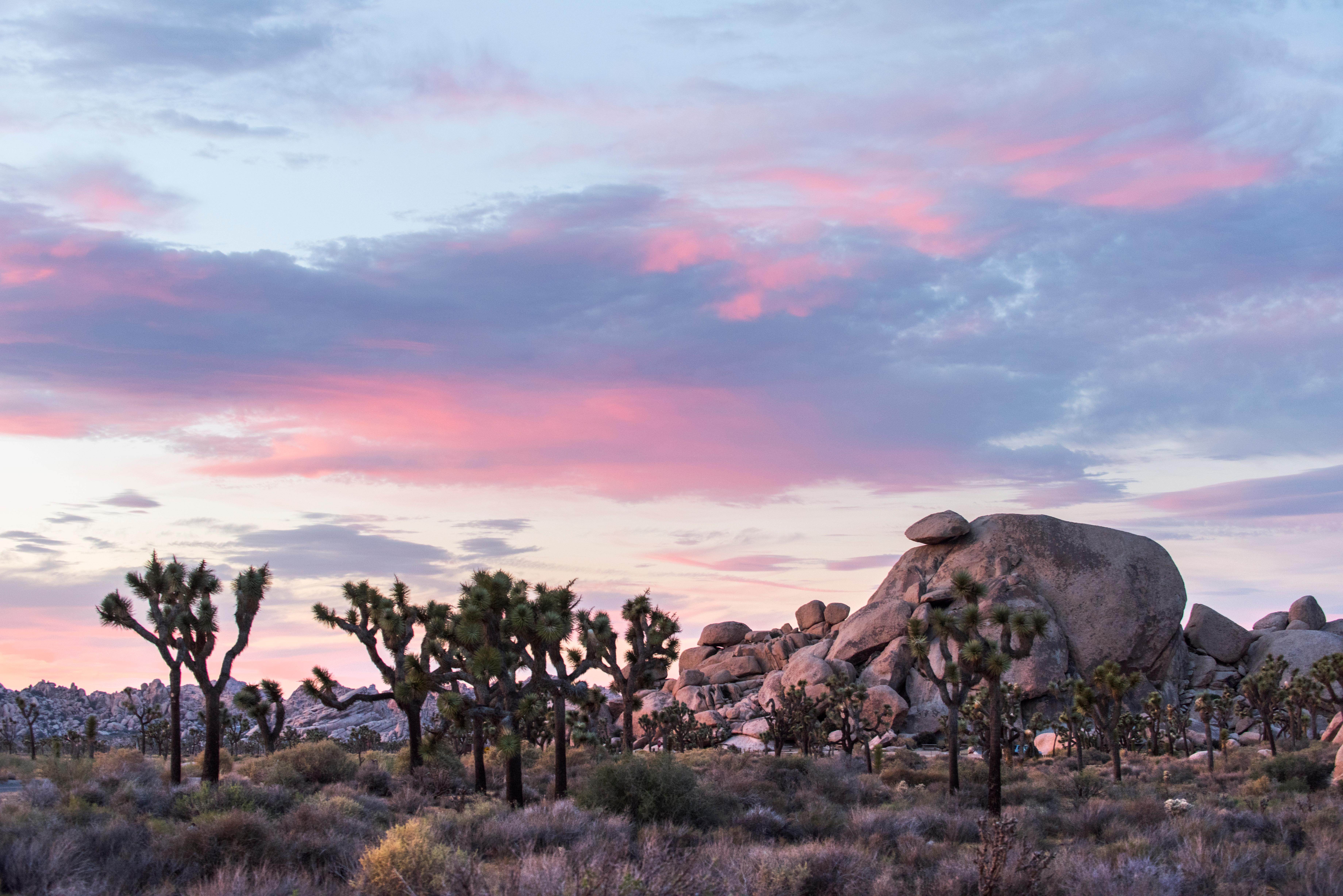This vividly detailed photographic artwork, with a photographic style that evokes the feel of a painting, captures the serene beauty of a sunrise at Joshua Tree National Park. In the foreground, a dense layer of green bushes and shrubs spans across the landscape, providing a lush base for the distinctive Joshua trees. These cacti-like trees, numbering about ten, rise gracefully from the arid desert floor. Five or six of them dominate the center of the image, flanked by pairs on either side. Towering above the vegetation, these trees exhibit shades of green and brown, contrasting with their rugged surroundings.

In the middle right section of the composition, a large boulder is surrounded by smaller gray and brown rocks, forming a natural yet imposing rocky cliff backdrop. The cliffs stretch horizontally, their stoic presence echoed by the scattered Joshua trees that stand in front of them.

Above this desert tableau, the sky occupies nearly three-fourths of the image. A breathtaking gradient of light blue to deeper hues frames ethereal white clouds tinged with orange, pink, and purple, suggesting the photograph was taken at sunrise. The color variation is most intense in the lower left, hinting at the sun's imminent appearance. This magnificent sky enhances the tranquil and timeless quality of the desert landscape, highlighting the interplay between the earthy terrain and the celestial spectacle overhead.